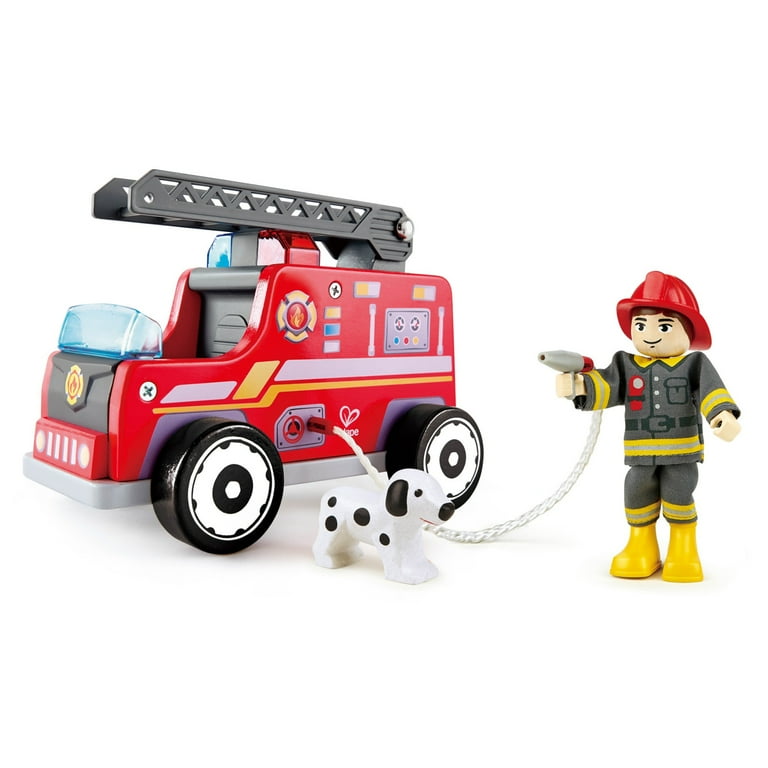The image depicts a classic Fisher-Price-style toy set featuring a vibrant red fire truck adorned with a gray ladder, detailed decals showcasing handles and gauges, and distinctive black and white wheels. The truck boasts a translucent blue plastic windshield and a similar blue piece atop it, simulating flashing emergency lights. In front of the fire truck stands an adorable white Dalmatian with black spots. Beside the dog, a firefighter minifigure dressed in a gray and yellow suit, yellow boots, and a red helmet, holds a fire hose connected to the truck, poised to respond to an imaginary blaze. The firefighter, a young boy with brown hair, adds a nostalgic touch, reminiscent of a favorite toy from childhood. The scene is meticulously staged, resembling a playful advertisement, evoking memories of timeless childhood adventures.